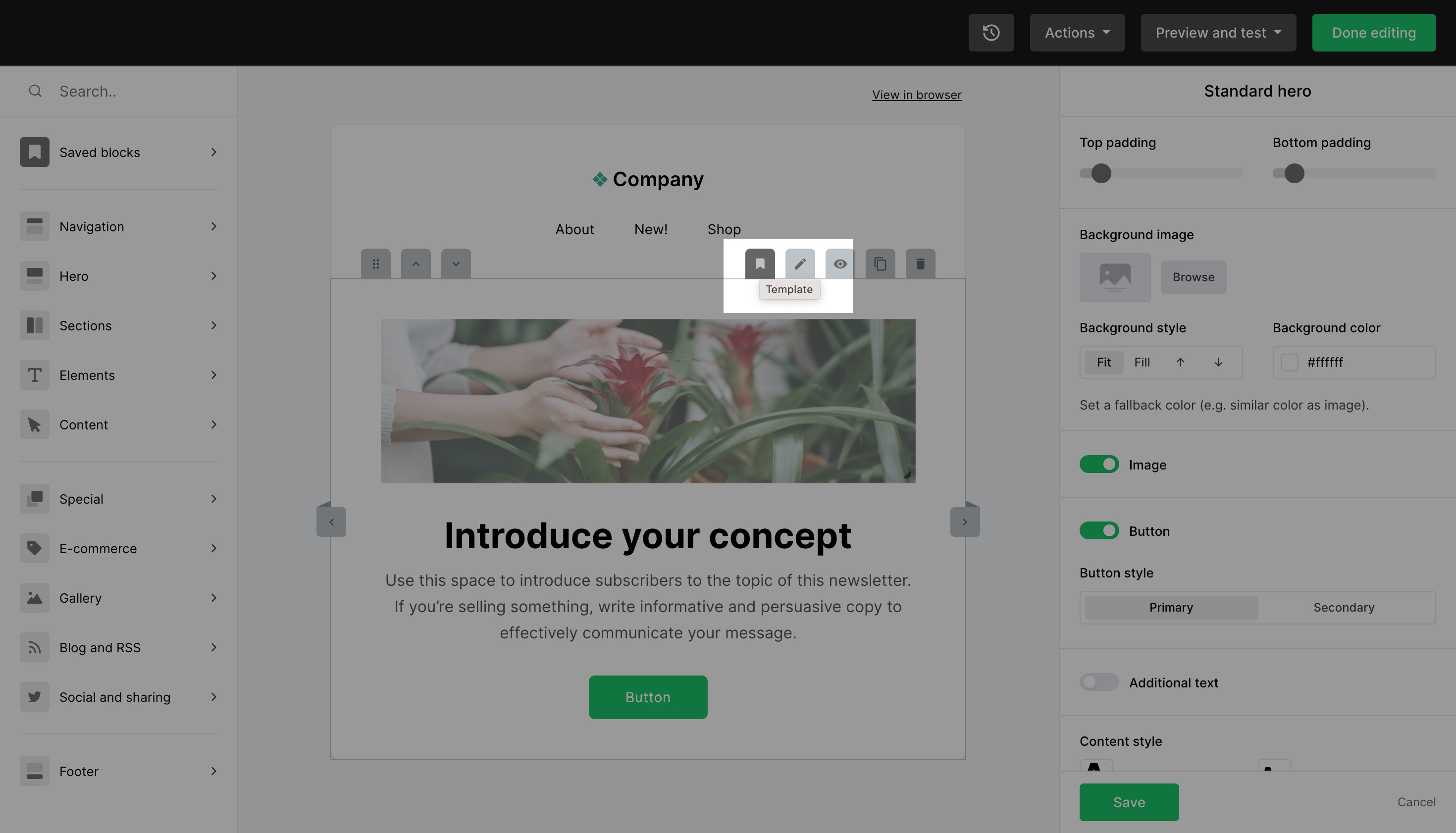The image showcases a grayed-out screenshot primarily highlighted with sections of white and black. The top portion features a black bar, while the right-hand side contains a gray square with navigational buttons, including "Refresh," "Actions," "Preview," and "Test." Notably, a green button with white text labeled "Done Editing" is prominently displayed.

The main body of the screen has a white background with a search bar in the upper left corner. Below this is a list of categories in black font: "Saved Blocks," "Navigation," "Hero Sections," "Elements," "Content," "Special," "E-commerce," "Gallery," "Blog and RSS," "Social and Sharing," and "Footer."

Within the gray-sided white screen, there is an image depicting Caucasian hands holding a green plant or flower from the left side of the frame. Above the image, "Company" is written in black. Below, the text reads, "Introduce your concept. Use this space to introduce subscribers to the topic of this newsletter. If you're selling something, write informative and persuasive copy to effectively communicate your message." Underneath this, there's a green square button with the word "Button" in white text.

At the top, there's a white-highlighted section labeled "Template," showcasing icons of a bookmark, a pencil, and an eye. On the right-hand side, several options for hero section customization are available, including "Top Heading," "Bottom Heading," "Background Image," "Background Style," "Background Color," "Image Button," and two buttons labeled "Save" and "Cancel" at the bottom-right corner.